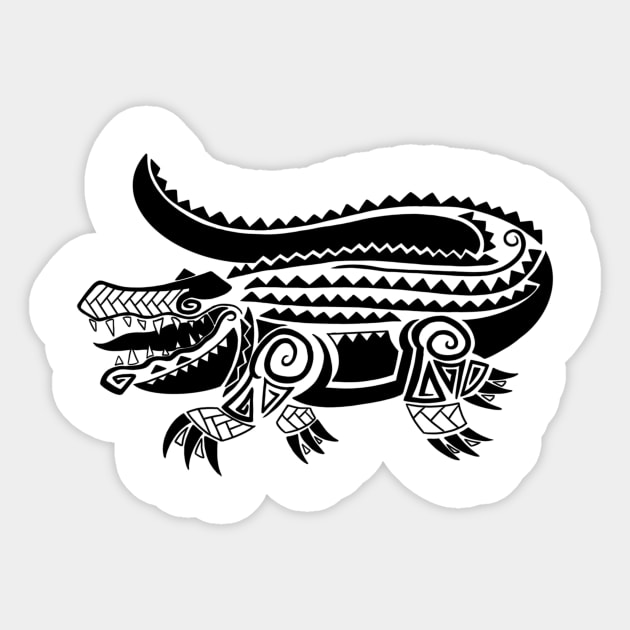This is an illustration of a black and white crocodile or alligator, rendered in a stylized, tribal art style reminiscent of Aztec designs. The creature's form is composed of bold, thick black lines with a stark white background. The simplicity is contrasted with intricate details; the back and tail feature numerous triangles, and the legs are constructed from a combination of rectangles and triangles for claws. The creature's face, assembled from interlocking trapezoidal shapes, is marked by a long, squiggly line that forms its mouth. Inside the open mouth, you can see two rows of roughly drawn, floating triangular fangs, lacking drawn gums, that surround the black tongue which ends at the front of the mouth. The entire artwork appears to be a sticker, characterized by a very bold and thick white border that cuts out the shape of the creature. This sticker sits on a pinkish-peach background, giving the appearance of clip art due to its overall composition quality.